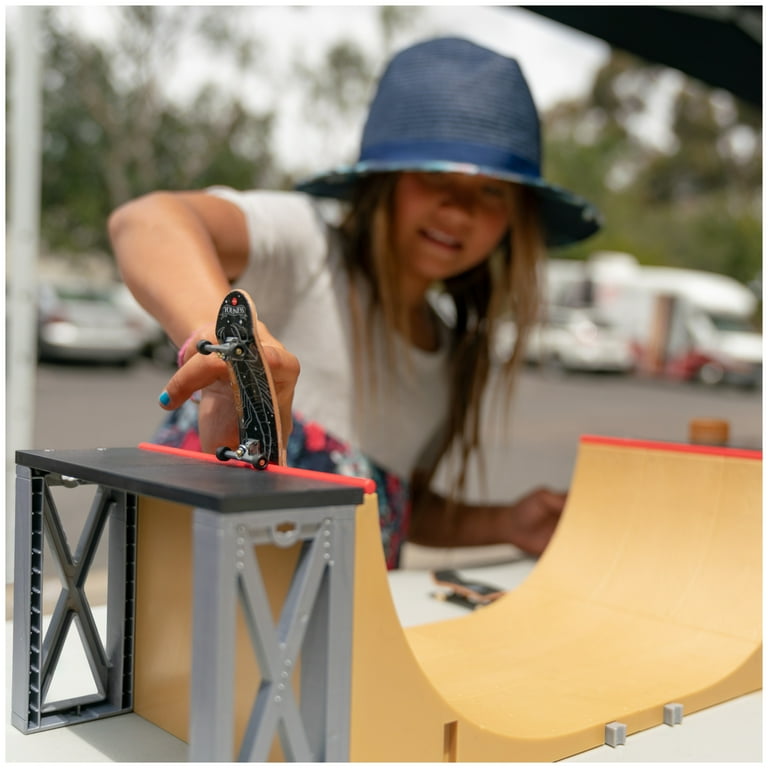In the photograph, a girl is intently playing with a finger skateboard on a tan-colored toy half-pipe. Her focus is on performing a lip trick at the edge of the half-pipe. The half-pipe features a support stand with rectangular legs designed with X-shaped crisscrosses and reddish tips. The girl, with her brownish-blonde hair partially covered by a blue hat, is wearing a white shirt with distinct blue, pink, and white trim at the bottom. Only one of her fingers is clearly visible, adorned with blue nail polish, while the rest are hidden by the finger skateboard, which is black with a scorpion design on it. The girl's face and body are slightly out of focus, drawing attention to her intricate maneuver on the finger skateboard. In the blurry background, there is a parking lot filled with cars and a camper, bordered by a line of trees under a gray daytime sky.